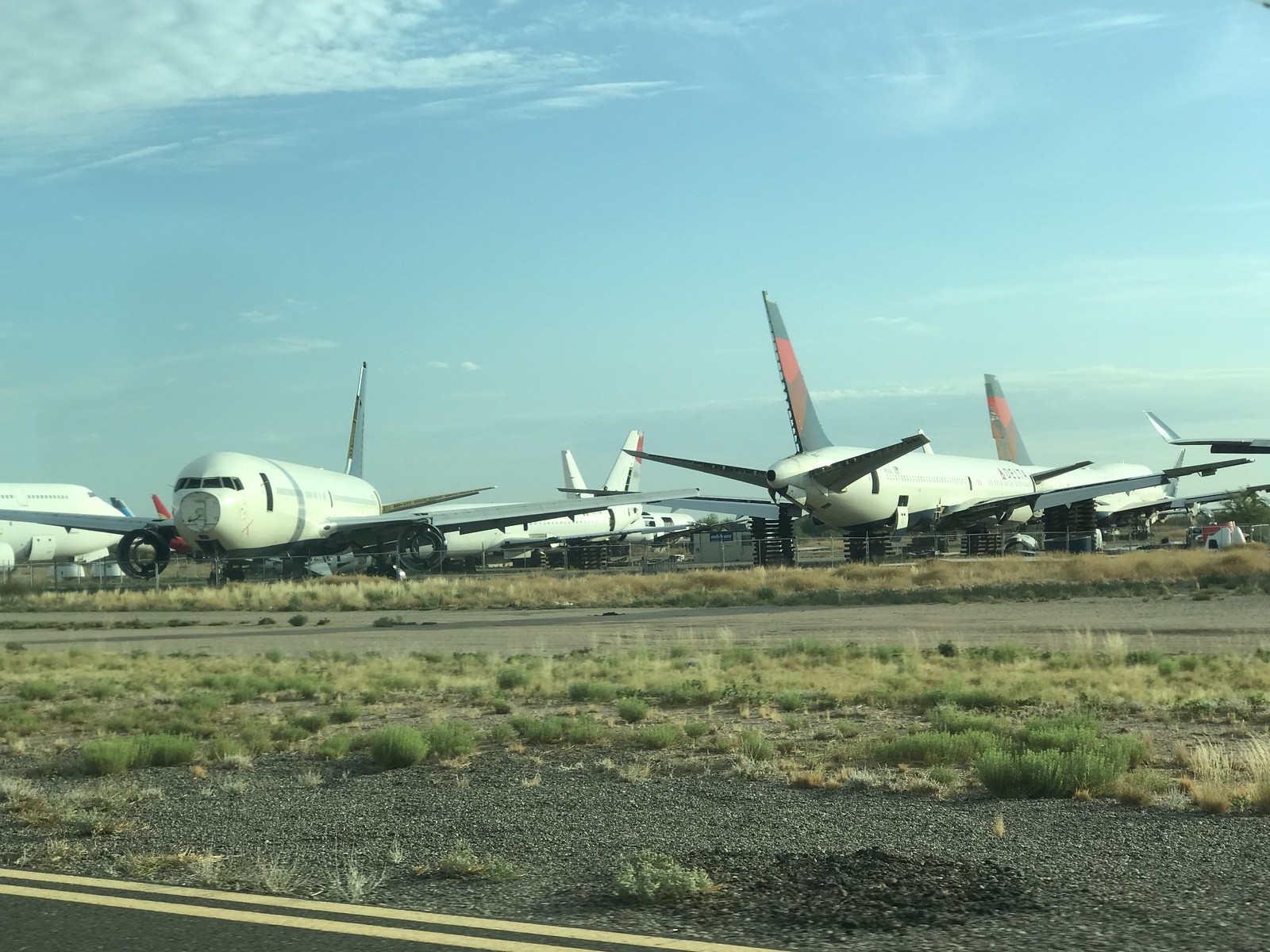The image captures a detailed scene of an airport boneyard, where large passenger airliners are parked in a somewhat haphazard arrangement. In the foreground, a rundown runway with faded yellow lines is surrounded by a gravel road, patches of loose grass, and a lot of dirt. The area appears neglected, with dying grass and weeds scattered around. Further back, five airplanes, some facing forwards and others backwards, are stationed side-by-side. All airplanes are white with gray wings and feature a red logo design; a few are identifiable as Delta Airlines planes, possibly Boeing 767s, with varying conditions. One aircraft notably has its nose combed out and engines removed. In the distant background, a hangar-like building can be seen under a bright blue sky, with light cirrus clouds and a misty mountain horizon adding to the isolated, almost desolate atmosphere of this storage area, reminiscent of places like the Marana in Arizona or Victorville in California.